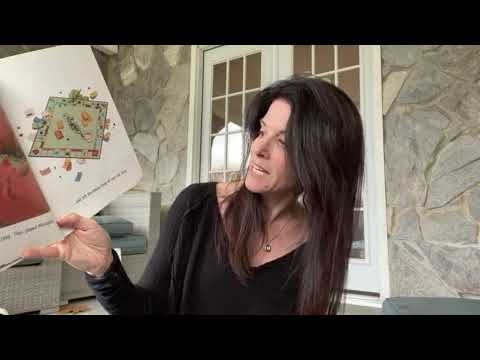The image depicts a thin, middle-aged Caucasian woman with long dark brown hair, seated in what appears to be a bright, stone-walled room with white doors and patio furniture. The furniture is made of white wicker adorned with dull teal pillows. She is wearing a black long-sleeved dress and a delicate necklace with a gold ring around her neck. The woman is deeply engrossed in reading a picture book, which she holds open with her right hand so the camera can capture its illustrations. The room is lit with natural daylight. She appears to be presenting or reading the book as she holds it up, possibly for an audience not visible in the image. Although the text in the book is blurry and indistinct, the page prominently shows what looks like a board game, perhaps Monopoly. The camera captures her engaged and thoughtful expression as she looks at the book. The image is framed with long horizontal black bars at the top and bottom.